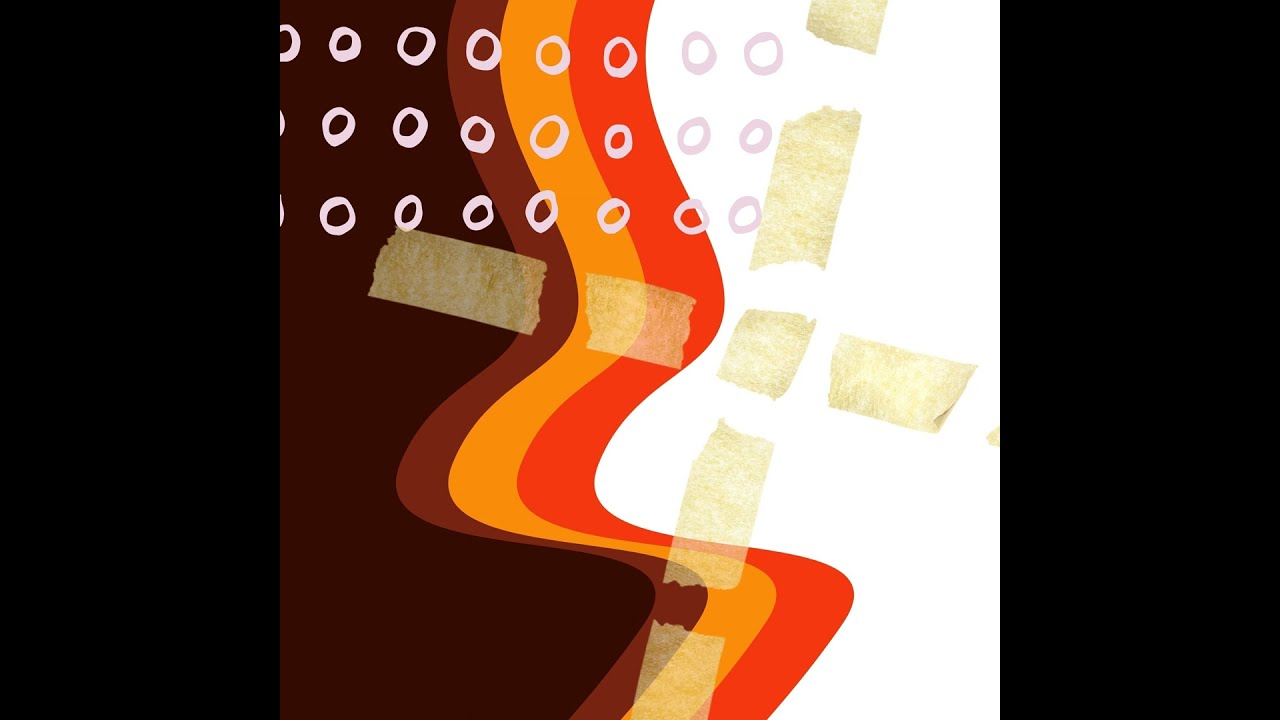The image is a landscape-oriented piece with wide black vertical borders on either side. In the center, a predominantly brown background transitions into white, framed by curving stripes of light brown, yellow, and orange. These stripes meander downwards, curving right, then left, sharp right, and finally back left, creating a vivid wave-like pattern. The top left corner features three rows of approximately eight hand-drawn, white circles—though some circles on the left are partially cut off.

In the middle section, a slightly diagonal cross is formed using eight pieces of masking tape with spaces between, converging around a central square piece of tape. Additionally, the tape appears torn in places, enhancing the cross shape with a rugged, improvised look. The entire composition, abstract in nature, may evoke commercial imagery through its color scheme and layout, resembling a stylistic advertisement devoid of text.